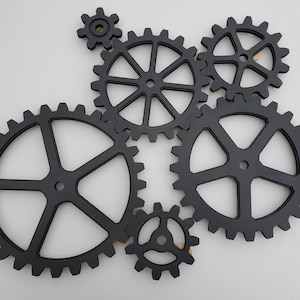This image presents a fascinating display of an abstract art installation featuring an intricate arrangement of interlocking gears mounted on a stark white wall. Each gear, meticulously painted in shades of black and monochrome grey, varies in size, contributing to the dynamic complexity of the composition. The gears are positioned to touch one another, suggesting a potential for motion where a single turn could set all the gears into synchronized movement. The diverse sizes range from extra small gears, such as a tiny one located in the top left corner, to very large gears dominating the lower section of the image. Medium-sized gears fill the spaces in between, creating a cohesive and visually engaging artwork. The minimalist white background accentuates the mechanical elegance of the gears, ensuring that they remain the focal point of the piece. The absence of any other objects emphasizes the intricate interplay and potential functionality of this captivating assembly.